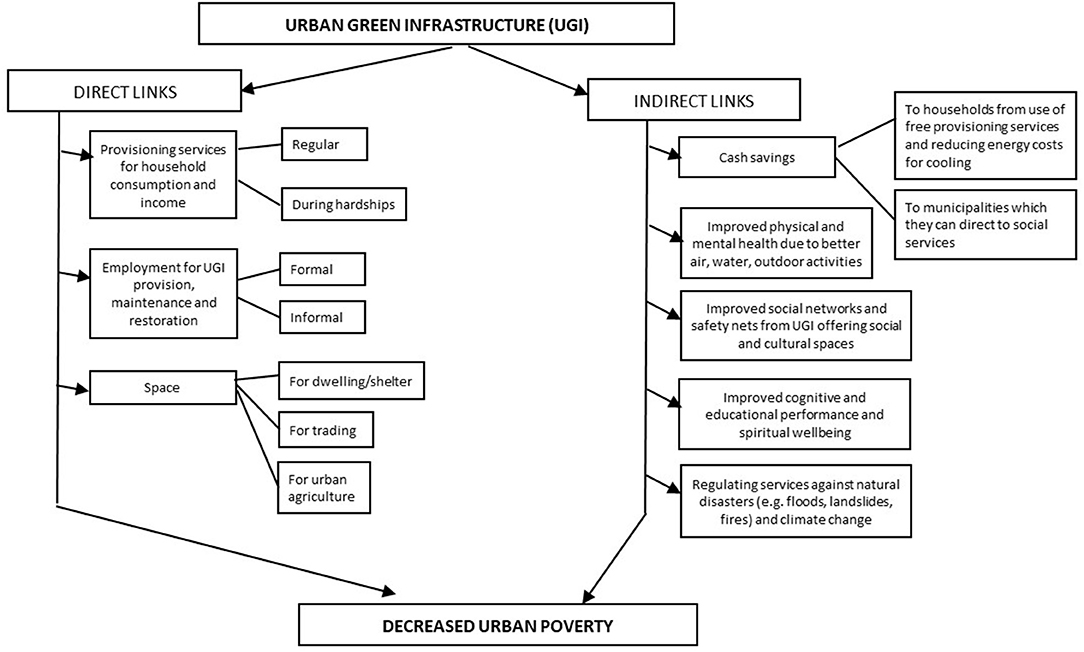This black and white diagram illustrates how Urban Green Infrastructure (UGI) can lead to decreased urban poverty. The image is arranged with various shapes—primarily rectangles of different sizes—and features text and arrows that map out both direct and indirect pathways of influence. At the top center, a long rectangle labeled "Urban Green Infrastructure" branches out into two directional columns: "Direct Links" and "Indirect Links."

In the "Direct Links" column, boxes detail specific benefits such as "Cash Savings," "Provisioning Services," "Employment for UGI Provisioning," "Maintenance and Restoration," and "Space." Each of these benefits is depicted as having a direct impact on urban poverty reduction.

In the "Indirect Links" column, additional positive outcomes are listed, including "Cash Savings," "Improved Physical and Mental Health," "Improved Social Networks," "Improved Cognitive and Educational Performance," and "Regulating Services Against Natural Disasters." Some of these outcomes have further sub-categories, exemplifying the nuanced benefits of UGI.

At the bottom of the diagram, a rectangle labeled "Decreased Urban Poverty" is connected by arrows to both the "Direct Links" and "Indirect Links" columns, signifying that all listed factors collectively contribute to reducing urban poverty. The entire diagram is rendered in black text against a white background, creating a clear and organized visual representation of how urban green infrastructure can systematically alleviate urban poverty.